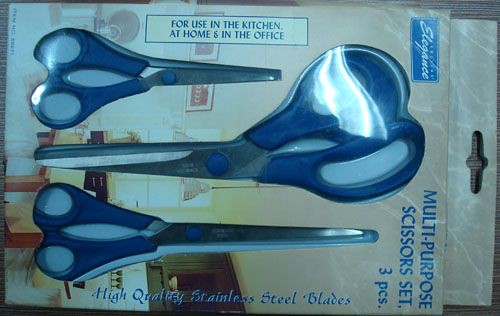This is a detailed photograph of a package containing a set of three multi-purpose scissors by the brand Elegance. The image is taken with the package turned sideways, revealing the text in blue font that reads, "Multi-purpose scissor set, three pieces." The package states that the scissors can be used in the kitchen, at home, and in the office, and highlights their "high quality stainless steel blades." The scissors feature blue handles and silver blades, with the Elegance logo prominently displayed in blue and white. The background of the packaging includes a neutral brown color with scenes that suggest different settings where the scissors can be used, like a kitchen or an office. The blister pack contains three pairs of scissors of varying sizes: a very long pair at the bottom, a standard-sized pair in the middle, and a smaller pair at the top, all within the unopened packaging. The image also captures some glare on the packaging, adding a realistic touch to the photo.